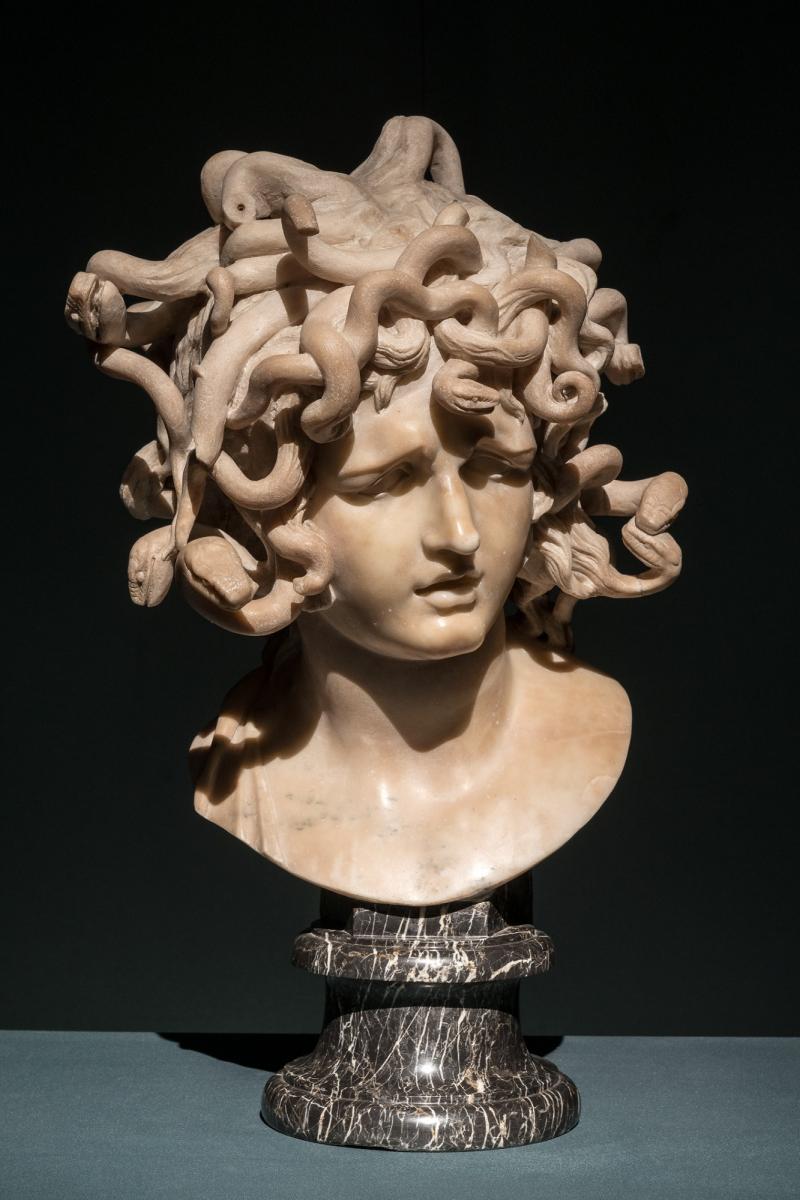The image captures a close-up photograph of a statue, specifically a sculpture of Medusa from Greek mythology. Only the head and neck of the sculpture are visible, and it prominently features hair made entirely of intricately carved snakes, with several snake heads distinctly visible on both sides of the head. The face of Medusa is detailed with carved-out eyes, a slightly open mouth, and a strong, almost masculine appearance.

The sculpture itself seems to be made from a smooth, light-colored stone, possibly marble, with hues of beige and darker browns adding texture. The Medusa head sits on a small, elegant pedestal crafted from grey granite with white streaks running through it. The pedestal features a round base that tapers upwards, composed of multiple disc sections. This entire piece is centered in the photograph, set against a dark grey and blue background that contrasts with a lighter blue floor, enhancing the sculpture's striking features.